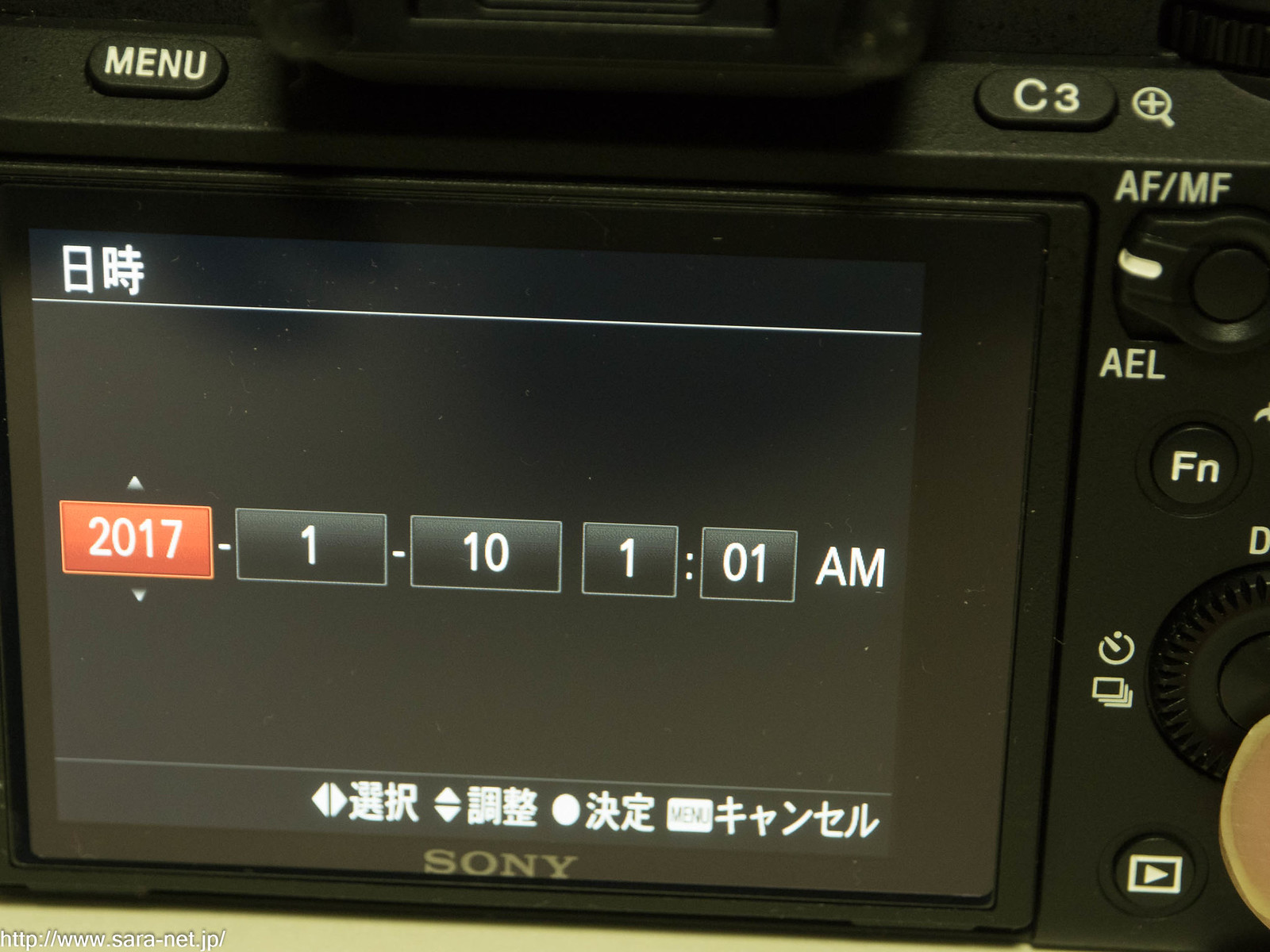This close-up image captures the intricate interface of a Sony digital camera. The device, which is black and square, features a flat screen with Chinese characters displayed, indicating a date and time setting. Prominently, the year "2017" is highlighted in a red box on the left side of the screen, followed by segmented sections showing "01:10:01 a.m." Below the screen, the Sony brand name is clearly visible. On the top-left corner of the camera, there is a MENU button, and on the top-right, a C3 button. The right side of the camera’s interface is crowded with several functional buttons and a dial. These include an AEL button, an AF/MF switch, an FN button near the center, and a play button depicting a square with a triangle inside, located at the bottom. Additionally, the screen's bottom left features a watermark with the URL "http://www.saranet.jp," adding a final touch to this detailed visual representation of the camera's features.